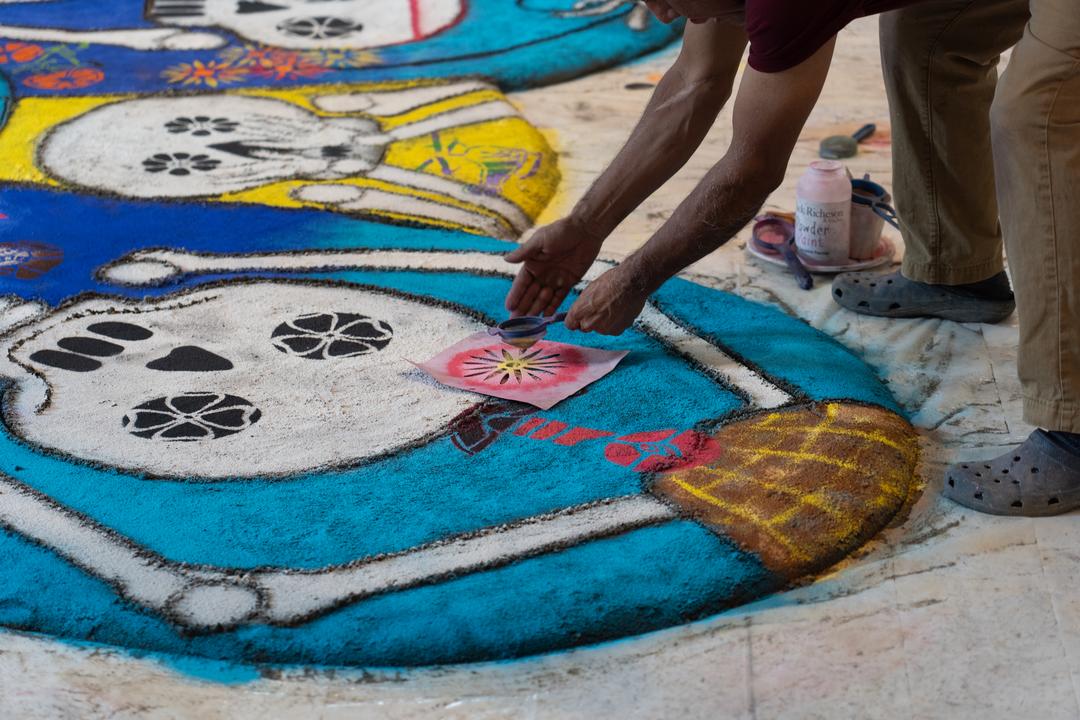In this detailed image, a brown-skinned man, dressed in light brown pants and dark-colored footwear—possibly crocs or flip-flops—is positioned on the right side. He is leaning over an intricately designed oval rug, which features various colors and patterns. The rug has a predominant blue hue with a darker segment towards its upper left center. It also contains a distinct brown portion to the right center adorned with brown and yellow squares, a white inner border running along its sides, and a white central area. The man appears to be carefully applying some drops of paint or colored sand onto the blue section of the rug through a stencil, which is placed atop the art piece. He is using a small sifter in one hand and tapping it with the other to distribute the material. The scene suggests this artwork is created using stencils, hinting at a possible cultural or ritual significance, reminiscent of colored sand art associated with Day of the Dead celebrations. Nearby, there is another rug in yellow, featuring similar symbolic designs and extensions from the right.